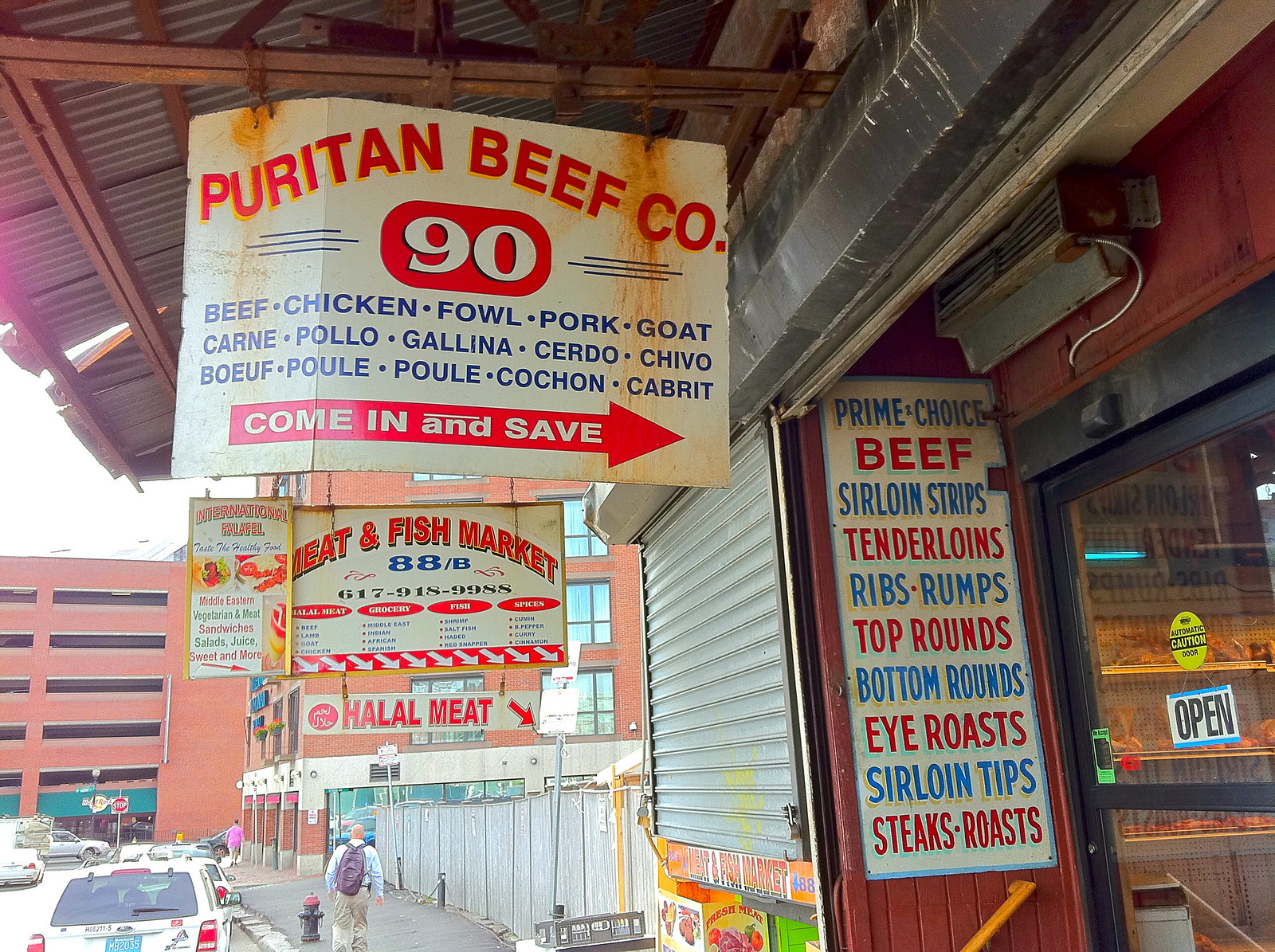The image captures the weathered storefront of Puritan Beef Company, which features a redwood facade and an awning supported by wooden rafters. The storefront includes a glass door marked with a "Caution" notice and an "Open" sign. To the left of the door, there is a detailed sign listing various meat products such as prime choice beef, sirloin strips, tenderloins, ribs, rumps, top rounds, bottom rounds, eye roasts, sirloin tips, and steak roasts, written in alternating red and blue fonts.

Above the entrance, an old cardboard sign prominently displays the company's name, "Puritan Beef Co." The number '90' is set in white font within a red oval, and beneath that, in blue text, it reads: "beef, chicken, fowl, pork, goat, carne, pollo, galena, churrito, chivo, boif, boulet, foulet, torchon, and cabret." A red arrow adjacent to this text points towards the right with the phrase "Come in and save."

The storefront also has a roll-up covering over a central window under the eaves. In the background, a building with a sign for "Halal Meat" can be seen, along with a few parked cars. The color palette includes shades of brown, red, white, blue, green, turquoise, yellow, and orange, indicating a vibrant setting outdoors in the middle of the day. The overall scene depicts a busy meat market area.